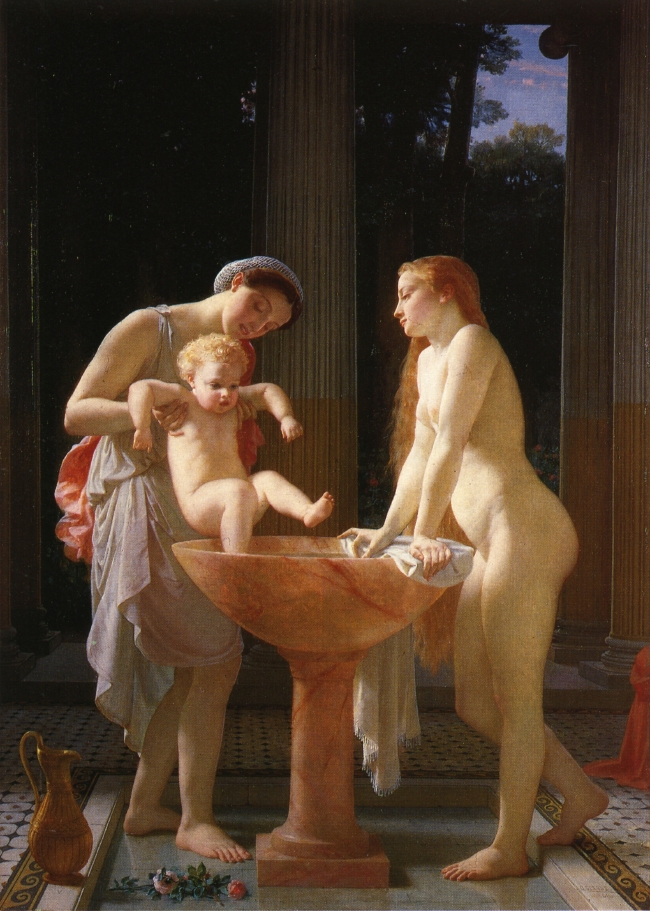This detailed painting, blending characteristics from the Renaissance and medieval eras, illustrates a serene indoor scene framed by classical architecture. At the center stands a tall, marble-like water basin, richly colored in shades of orange and red, where a naked baby with blonde, curly hair is being bathed. To the left, a woman draped in loose, classical attire featuring a white toga and pink coverings, holds the baby. Her brown hair is pulled back in a blue bonnet. Beside her, a gold pitcher rests near the basin’s edge.

To the right, another woman, fully nude, leans over the basin with her hands clasped on its rim. She is curvaceous and has extraordinarily long, cascading red hair that falls nearly to her knees. The ornate floor beneath them is a regal checkered pattern of black and yellow marble.

The background is adorned with imposing white marble columns tinged with orange hues at their bases, contributing to the grandeur of the scene. It appears to be dusk, with a darkening forest silhouetted against the fading light and a sky streaked with hints of blue and white puffy clouds. The overall atmosphere evokes a timeless ritualistic scene, rich with cultural and historical undertones.